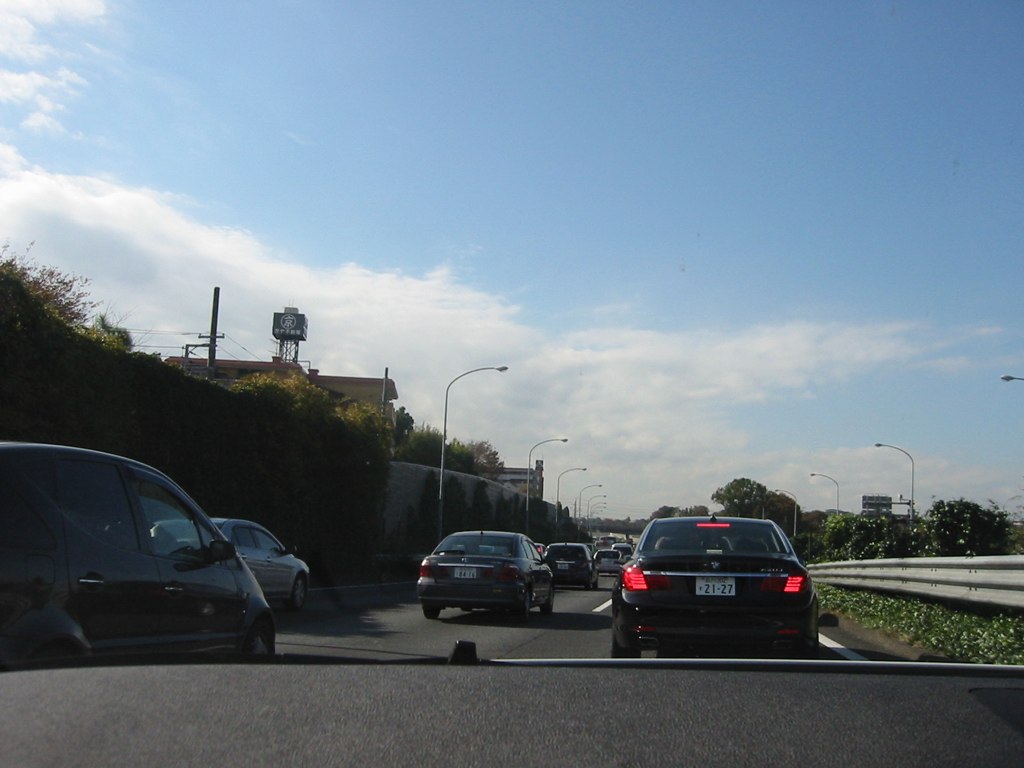This square-shaped image captures an outdoor scene featuring a road bustling with traffic. The sky overhead is a light blue adorned with scattered clouds. The road spans three lanes, each filled with cars moving forward. On the right side, a silver guardrail runs parallel to the lanes, with green grass and lush plants growing below and extending into the background. The backdrop is punctuated by green trees, creating a serene natural frame for the scene. Streetlights are positioned on both sides of the road, further enhancing the depth and perspective of the image.